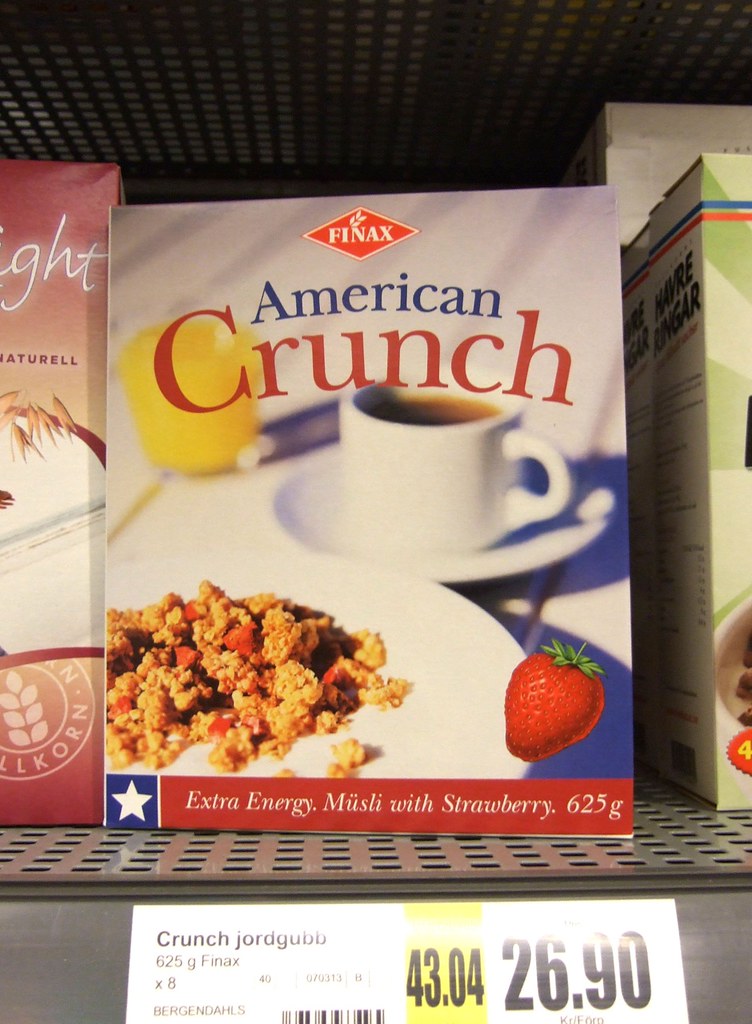The image depicts a grocery store aisle containing a shelf with a prominent cereal box. The box, labeled "American Crunch," features bold red, white, and blue colors. At the top, "FINAX" is printed in white within a red diamond shape. The box showcases various visual elements: a white coffee cup filled with coffee on a white saucer, a short glass of orange juice, and a white bowl of muesli cereal in the foreground. A ripe strawberry with a green stem sits at the bottom right of the bowl. The bottom of the box features the text "Extra Energy Muesli with Strawberries, 625 grams," printed on a blue background with a white star to its left. Directly below the box on the metal shelf, a white label reads "Crunch JORDGABB" alongside price indicators "43.04" in black on a yellow square and "2690" to the right. The shelf and parts of the store's gray ceiling, both featuring holes, are visible, along with hints of other cereal boxes adjacent to the American Crunch box—pinkish on the left and white and brown on the right.